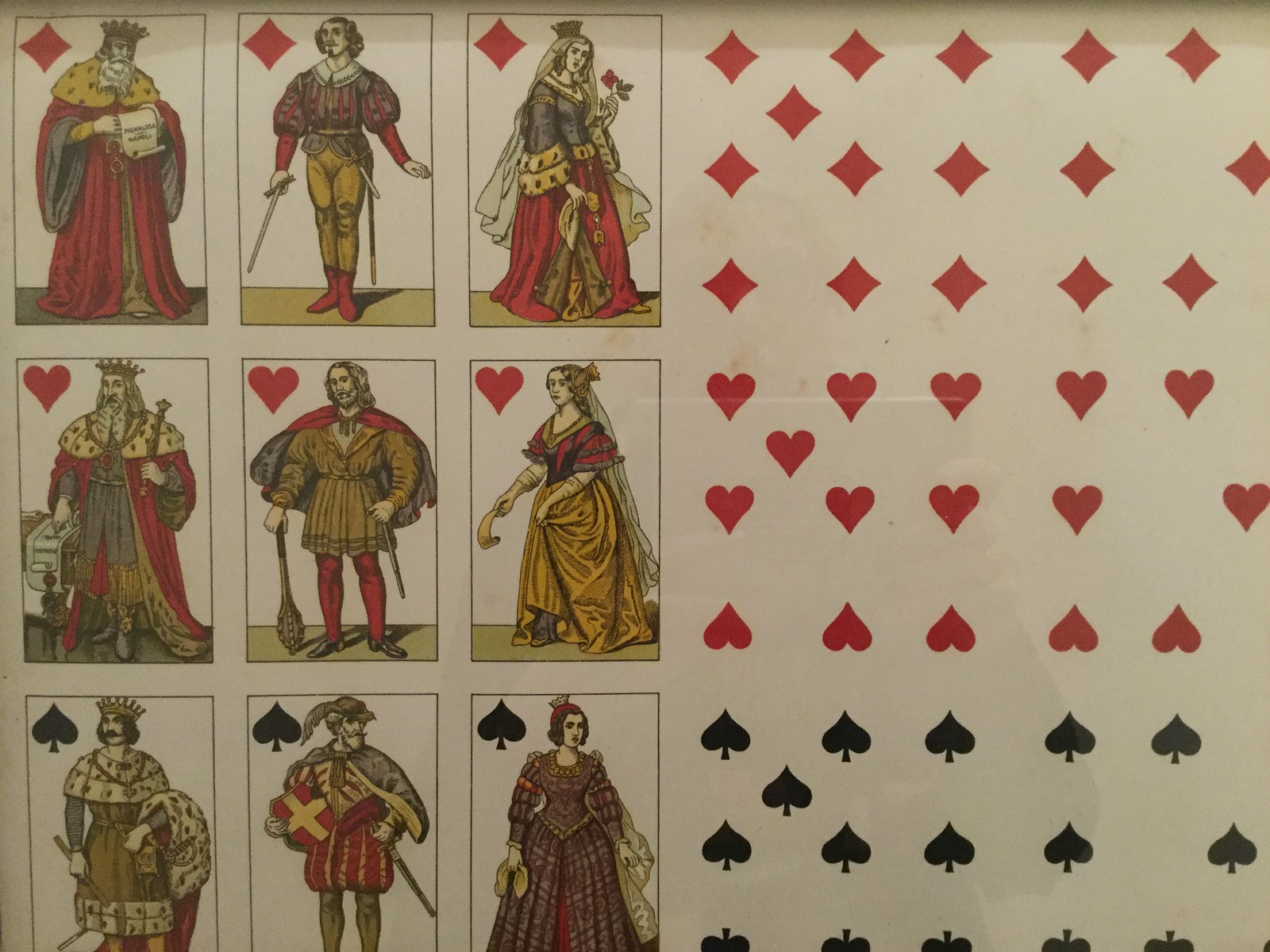This intricate illustration is a full-body artistic rendition of the traditional playing card figures, including a King, a Queen, and other familiar characters typically depicted on cards. Unlike conventional playing cards where only the upper half and a mirrored bust are shown, this detailed drawing captures each figure from head to toe. Alongside these regal and noble characters, the image features playing card symbols (suits) organized in three distinct rows: the top row displays red diamonds, the middle row shows red hearts, and the bottom row features black clubs. Each figure is uniquely associated with a specific row, indicating a correlation with the different suits. On the left side, the symbols are meticulously arranged in a descending order: five diamonds, four diamonds, and then three clubs at the bottom, each group clustered closely together. This vivid and comprehensive artwork brings a fresh, detailed perspective to classic playing card imagery.